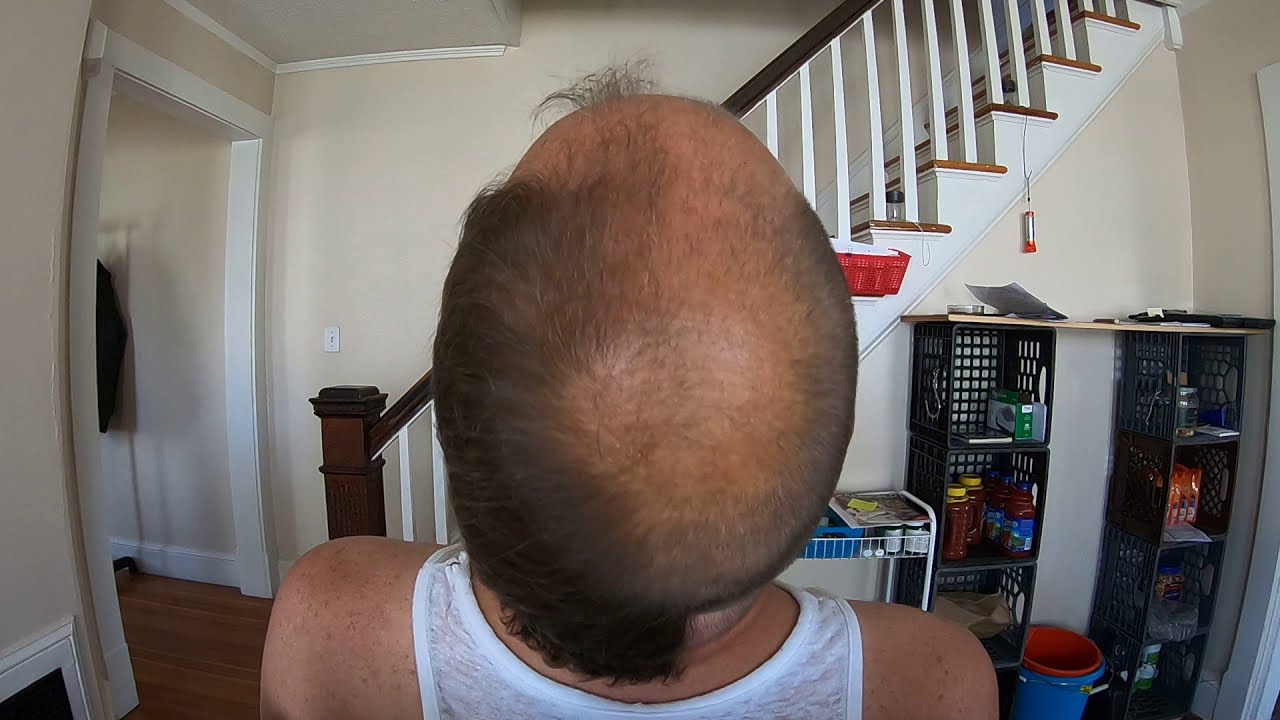This image captures the back of a man's head, emphasizing his partially shaved hair. The left side of his head retains its natural brown hair while the right side is closely shaved down to stubble, revealing a receding hairline and a large balding spot towards the crown. The man, wearing a white t-shirt, appears to be in the middle of self-grooming, possibly in his own house. The background features a white staircase leading upstairs, with wooden handrails. In front of the staircase are stacked milk crates filled with various office and food items, alongside a small white storage cart. To the left of the scene, a coat hangs on the wall, visible through an adjoining room's doorway. The overall setting suggests a casual, lived-in environment with practical storage solutions.